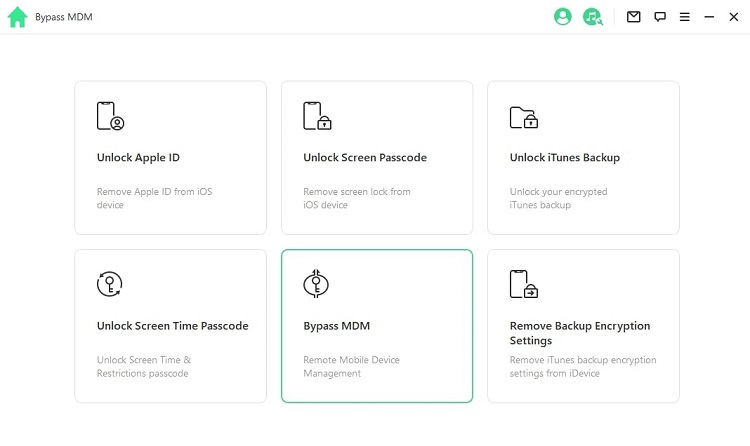The image displays a website interface. At the top left, there is an icon of a green house, followed by the text "Bypass MDM," with the first letter "B" and the letters "MDM" capitalized. Moving towards the right side, there is a graphic of a person inside a green circle. Adjacent to it, there is another circle containing a music note. Further right, there are several icons positioned in sequence: a small line, an envelope, a text bubble, three horizontal lines stacked together, a minus sign, and an "X."

Below these icons, a thin dividing line separates the top section from the white background below. Displayed on the white background are six equally-sized squares arranged in two rows of three. The text inside these squares reads as follows:

1. "Unlock Apple ID"
2. "Unlock Screen Passcode"
3. "Unlock iTunes Backup"
4. "Unlock Screen Time Passcode"
5. "Bypass MDM" – This square is highlighted with a muted greenish-blue color and a border around it.
6. "Remove Backup Encryption Settings"

Each square represents a different function related to device security and data management.